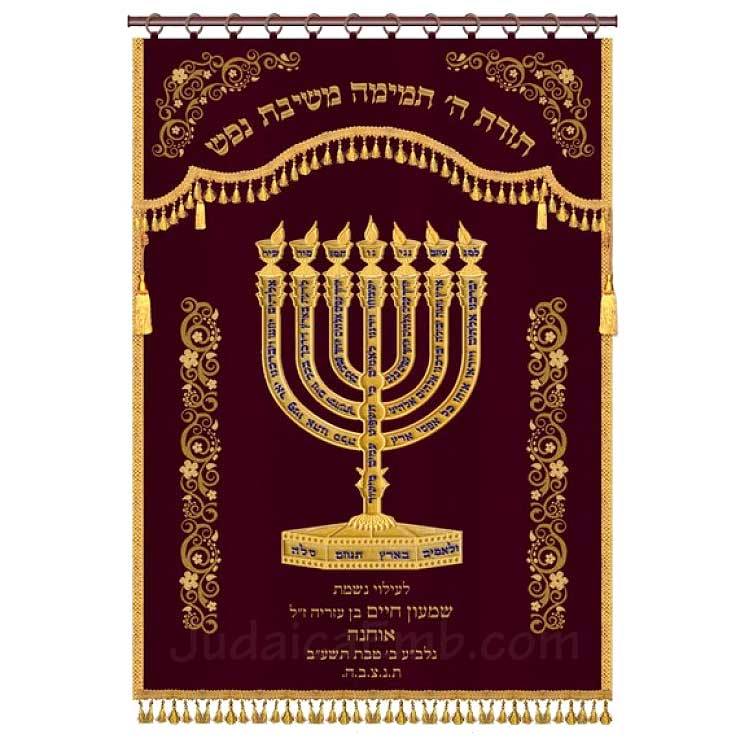The image depicts a vertically hanging, rug-like tapestry, taller than it is wide, approximately one and a half times its width. It is suspended from a dark red curtain rod with 12 circular rings. The tapestry is a rich maroon color, bordered on three sides (left, right, and bottom) with intricate golden embroidery. Its bottom edge features decorative gold tassels. The centerpiece of the design is a golden menorah with seven U-shaped candle holders. Surrounding the menorah and lining the edges of the tapestry are ornate designs of ivy, flowers, and swirls. Additionally, there is Hebrew text embroidered in gold at both the top and bottom of the tapestry.